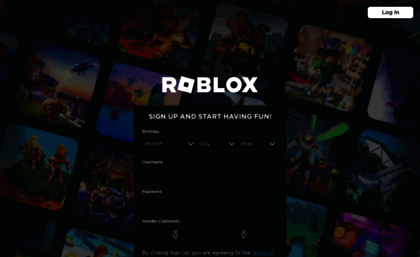This is a detailed screenshot of the Epic Games Store featuring the Roblox sign-up page. Dominating the screen is the signature Roblox logo, notable for its unique 'O' which is designed as a square box with a dot in the center. In the top right corner, there is a white "Login" button. Centered prominently on the page, a larger black box invites users to "Sign Up and Start Having Fun."

The registration form requires users to input their birthday through drop-down menus for the month, day, and year. Following this, there are fields to select a username, input a password, and choose a gender. At the bottom of the form, users must agree to the terms of service, which gets cut off in the screenshot.

The background is a dynamic mosaic of scenes from Roblox, including various in-game settings. One segment shows two characters standing on an island, gazing at a sunset under a partly cloudy sky. Another section features characters running with a helicopter flying overhead, among other vibrant screencaps reflecting different aspects of the game. The diverse imagery encapsulates the immersive and varied experiences Roblox offers its players.